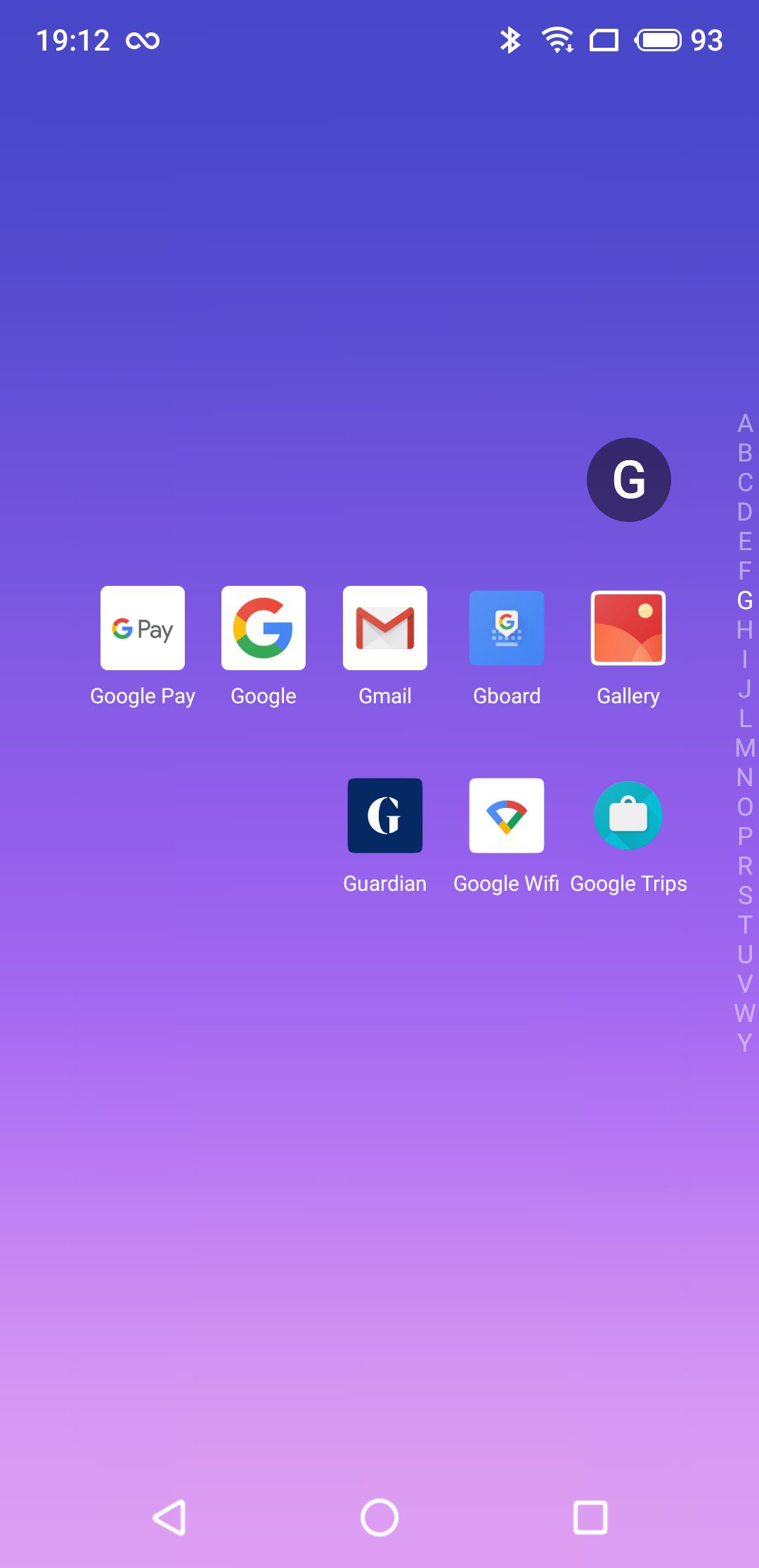The image depicts a homepage of a mobile phone. The status bar at the very top left displays the time as "19:12" in white, followed by an infinity symbol represented by two overlapping circles. The top right corner features several icons: a Bluetooth logo, signal bars indicating service strength, a symbol resembling a micro SD card with the top left corner cut out, and a battery icon showing a full charge with "93" percent next to it.

The background shows a gradient transitioning from dark purple at the top to a lighter shade towards the bottom. Centrally located, there are several application icons predominantly from Google. From left to right, the apps are organized as follows: 
- Google Pay
- Google
- Gmail
- Gboard
- Gallery
- Guardian
- Google Wi-Fi 
- Google Tips

In the top right corner of this section, there is a black circle containing a white "G." To the far right side of the screen, there are alphabetical shortcuts listed from "A" to "Y" in a grayed-out color with the "G" highlighted in white.

At the very bottom of the screen, there are three navigation buttons: a back button, a home button, and a square. All these buttons are in white, with the specific function of the white square on the bottom right being unclear.